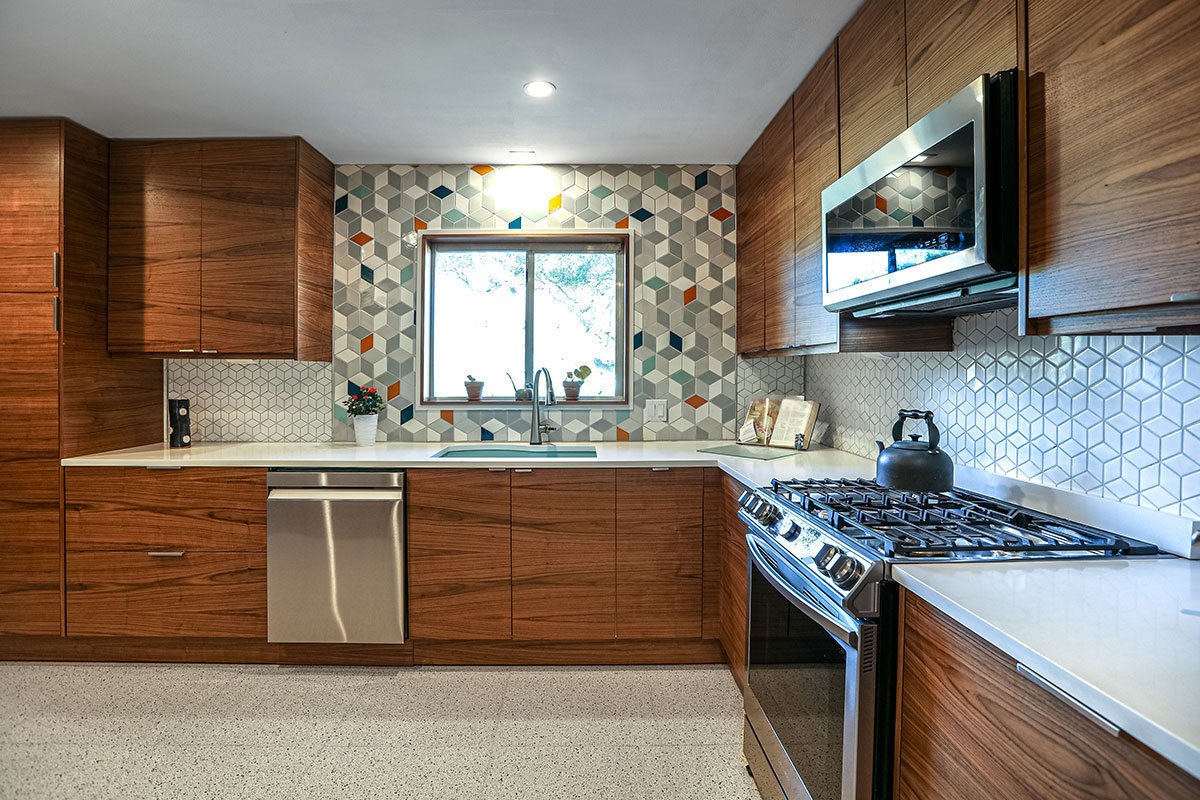This image captures a pristine kitchen, showcasing a meticulously clean and organized space that resembles a model kitchen shot. The kitchen features natural wood cabinets, highlighting the wood grain and equipped with metal handles, wrapping around from the bottom right of the photo up to the left side, covering the entire floor area. The countertops are made of a white granite-like material, accentuating the modern and sleek aesthetic.

On the right side of the photo, there is a modern stainless steel oven with a cast iron top, and above it, a microwave with a metal finish and black glass front. To the left, embedded within the cabinetry, is a stainless steel dishwasher. Additionally, there is a gas stove with a teapot placed on it, enhancing the kitchen's welcoming ambiance.

The backsplash features a striking geometric pattern of hexagonal tiles, in a mix of grey and white, with random injections of color such as reds, greens, oranges, and blues, adding a vibrant touch to the space. The white tile floors, speckled with a subtle design, coordinate perfectly with the kitchen’s chic and modern look. 

Situated next to a window, which offers a view of a few trees outside during the daytime, the kitchen is bathed in natural light, further elevating its inviting atmosphere.